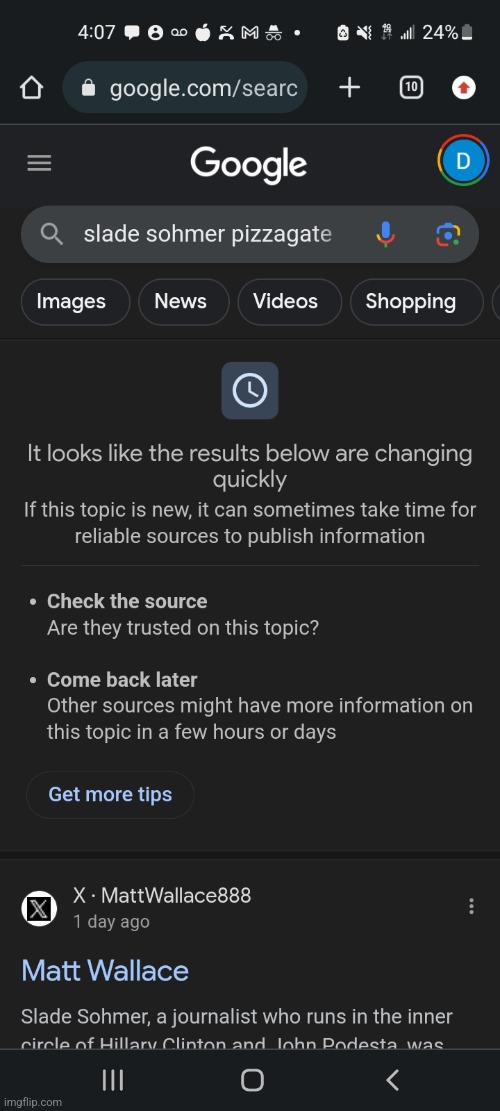The image displays a screenshot of Google search results for "Slayed Somer Pizza Game." At the top of the screen, the time displayed is 4:07, and a series of icons are present including the messaging and voicemail icons, a Gmail symbol, a missed call notification, and a cell phone reception icon. The battery level is at 24%.

Beneath this status bar is the Google search bar, followed by another search bar specific to web queries. Below these bars are tabs for various types of search results, including Images, News, Video, and Shopping.

Directly below these tabs, a message states, "It looks like the results below are changing quickly. If this topic is new, it can sometimes take time for reliable sources to publish information." There is further guidance advising users to "Check the source" and "Come back later" for more reliable information.